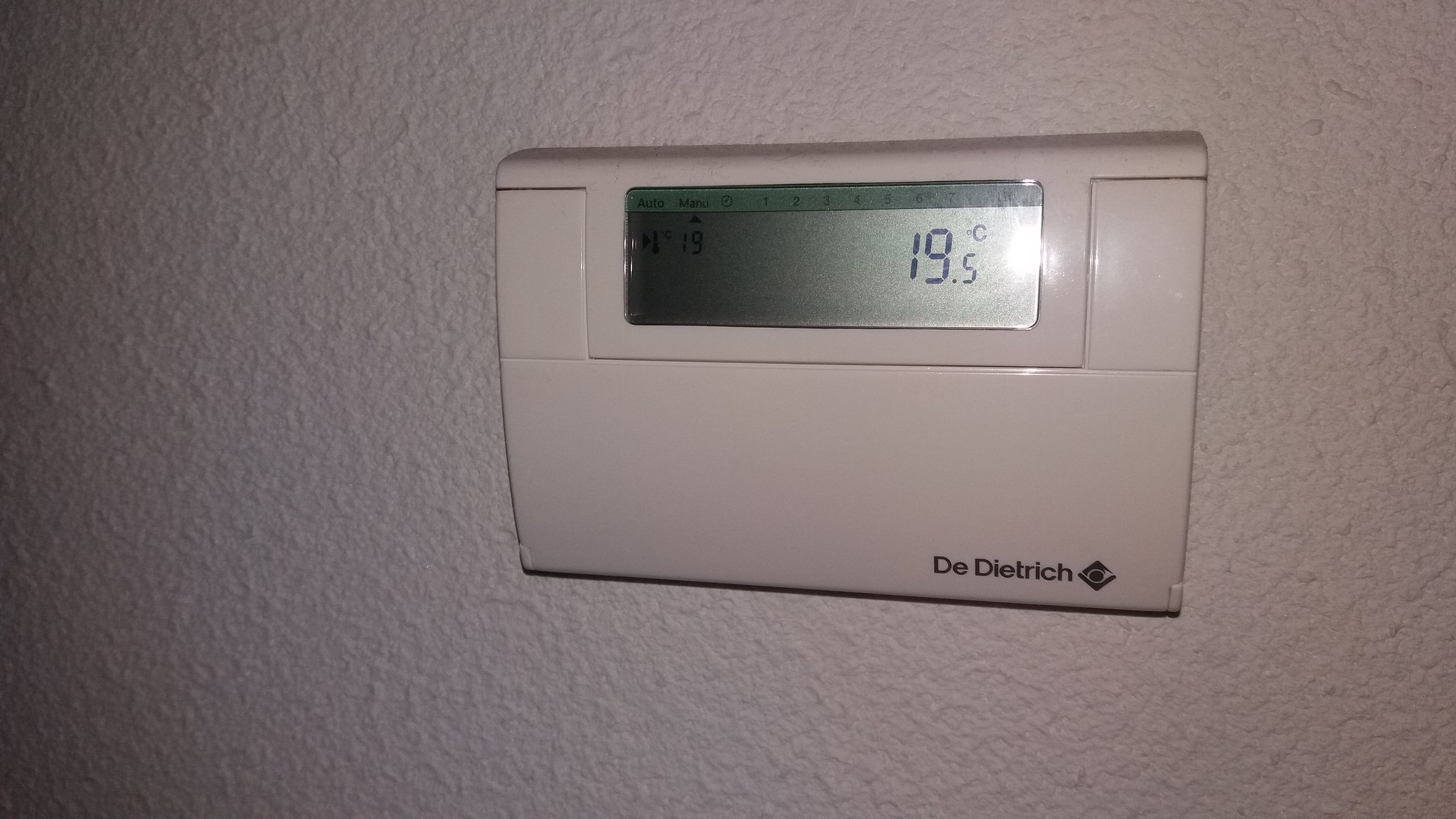The image portrays a white thermostat mounted against a white plaster wall adorned with small memos. The thermostat has a flip-top cover that opens, revealing a long screen at the top center which displays various details. The screen shows a temperature reading of 19.5 Celsius on one side, although a glare from the light obscures part of the display, making it difficult to read other details clearly. Despite this, the words "Auto" and "Matrix" can be discerned among the top indicators, along with symbols like an arrow, the number '1,' and 'Celsius.' The thermostat also bears the brand name "French VIETRICH" on the bottom of the flip-top cover. The lighting creates a blinding effect on the far side of the screen, leaving some sections blurry and unreadable.